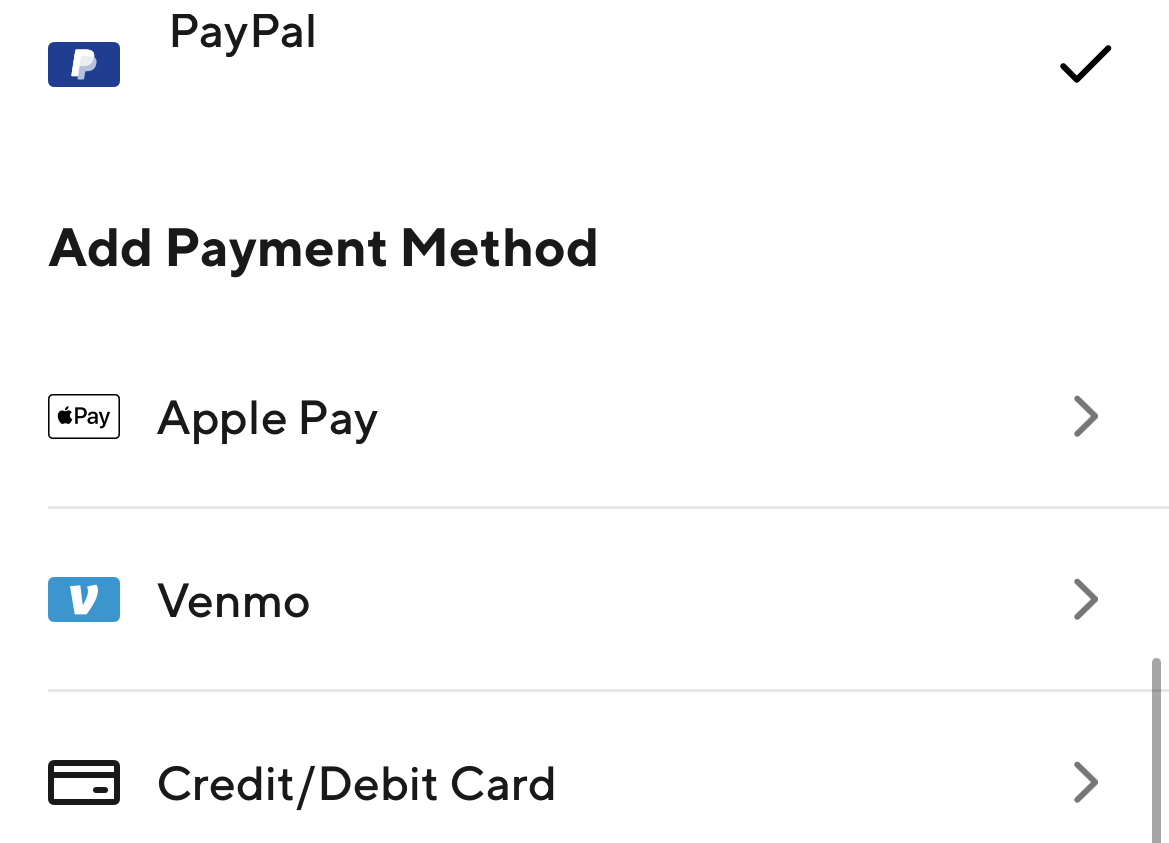A screenshot of a mobile payment methods screen showcasing options for a purchase. The interface has a clean, white background typical of a mobile device. At the top, there is the PayPal option featuring a small PayPal logo on the left and the text "PayPal" to its right. A checkmark on the far right of the screen indicates that PayPal has been selected as the current payment method. Below this, in slightly larger black text, is the option to "Add Payment Method."

Following the PayPal option, three additional payment methods are listed. The first is Apple Pay, accompanied by a small Apple Pay logo on the left. To the right, an arrow points to the right, suggesting that this option can be selected by tapping. Below Apple Pay is the Venmo option, with a small Venmo logo on the left and a similar arrow on the far right. The final payment option listed is "Credit/Debit Card," indicated by a small card logo on the left, with another right-pointing arrow on the far right, indicating it can be selected as well.